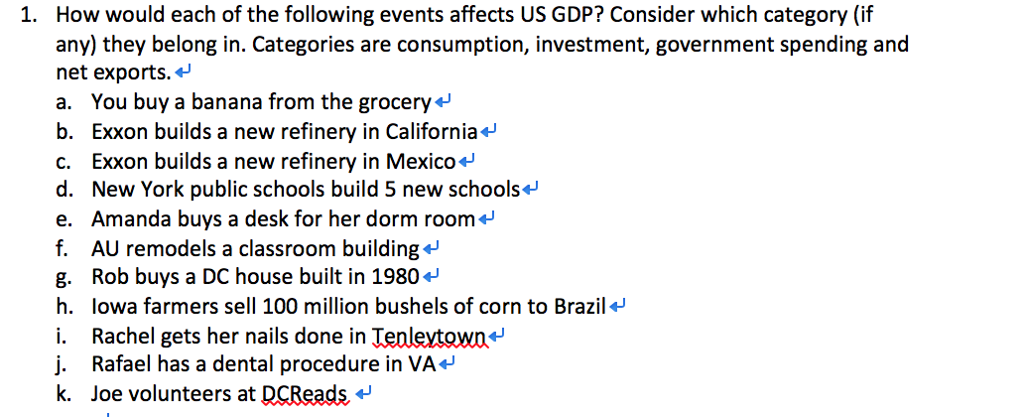This screenshot displays an entry on a white background with standard dark black or dark gray text. The title reads, "How would each of the following events affect US GDP? Consider what category, if any, they belong in." Categories include consumption, investment, government spending, and net export. The entry consists of a list of events, each accompanied by a blue, bent arrow pointing towards it. The events are as follows:

A. You buy a banana from the grocery.
B. Exxon builds a new refinery in California.
C. Exxon builds a new refinery in Mexico.
D. New York public schools build five new schools.
E. Amanda buys a desk for her dorm room.
F. AU remodels a classroom building.
G. Rob buys a DC house built in 1980.
H. Iowa farmers sell 100 million bushels of corn to Brazil.
I. Rachel gets her nails done in Tinleytown.
J. Raphael has a dental procedure in Virginia.
K. Joe volunteers at DC Reads.

This structured task list aims to prompt an analysis of how various events impact US Gross Domestic Product (GDP) by classifying each into the appropriate economic category.